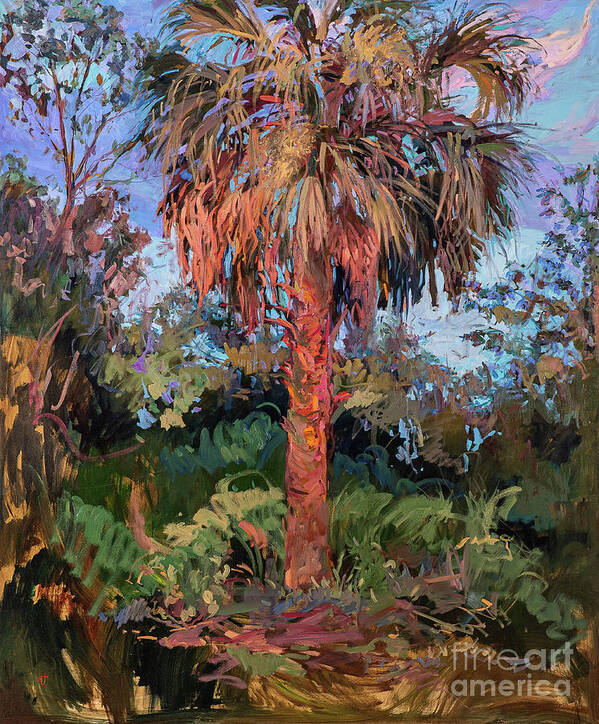In this rectangular artwork, potentially an oil painting or digital composition, the central focal point is a beautifully detailed palm tree with a trunk showcasing a blend of brown, green, grey, red, yellow, and pink hues. The top of the tree features vibrant green fronds interspersed with some brown, dying fronds at the bottom. The setting hints at a light forest or grove scene, especially on the left, which is denser with greenery, including a skinny branch tree accompanied by shrubs and bushes. On the right, the foliage is more subdued, with thin branches and fresh green leaves. The background sky is a psychedelic mix of blues, purples, and pinks, adding a surreal quality to the scene. Broad, undefined strokes characterize the foliage surrounding the base of the palm tree, creating an impressionistic feel with splashes of black, blue, green, cream, and brown. The painting bears a watermark in the lower right corner, indicating it is from Fine Art America.